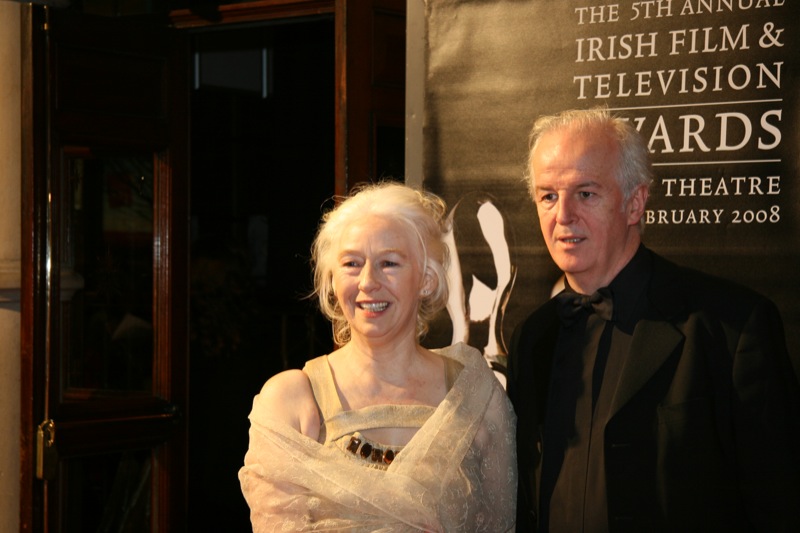The photograph captures an elderly couple in their late 60s or early 70s, standing together and posing for the camera at a special event. Both have white or gray hair, with the man appearing slightly balding, and the woman with her hair elegantly styled up. She is beaming a warm smile, while the man has a blank but pleasant expression. The woman is dressed in a light-colored dress adorned with a delicate lacy shawl draped over one shoulder, exuding an air of grace and sophistication. The man is attired in a black suit, complemented by a black button-down shirt and a black bow tie, completing his formal look. They are positioned in front of a backdrop, which features a black banner with white text that reads, "The 5th Annual Irish Film and Television Awards, February 2008." The scene appears to be set in the evening at a prestigious theater event, suggested by the presence of photographers and an inviting brown wooden door with glass panels visible in the background.